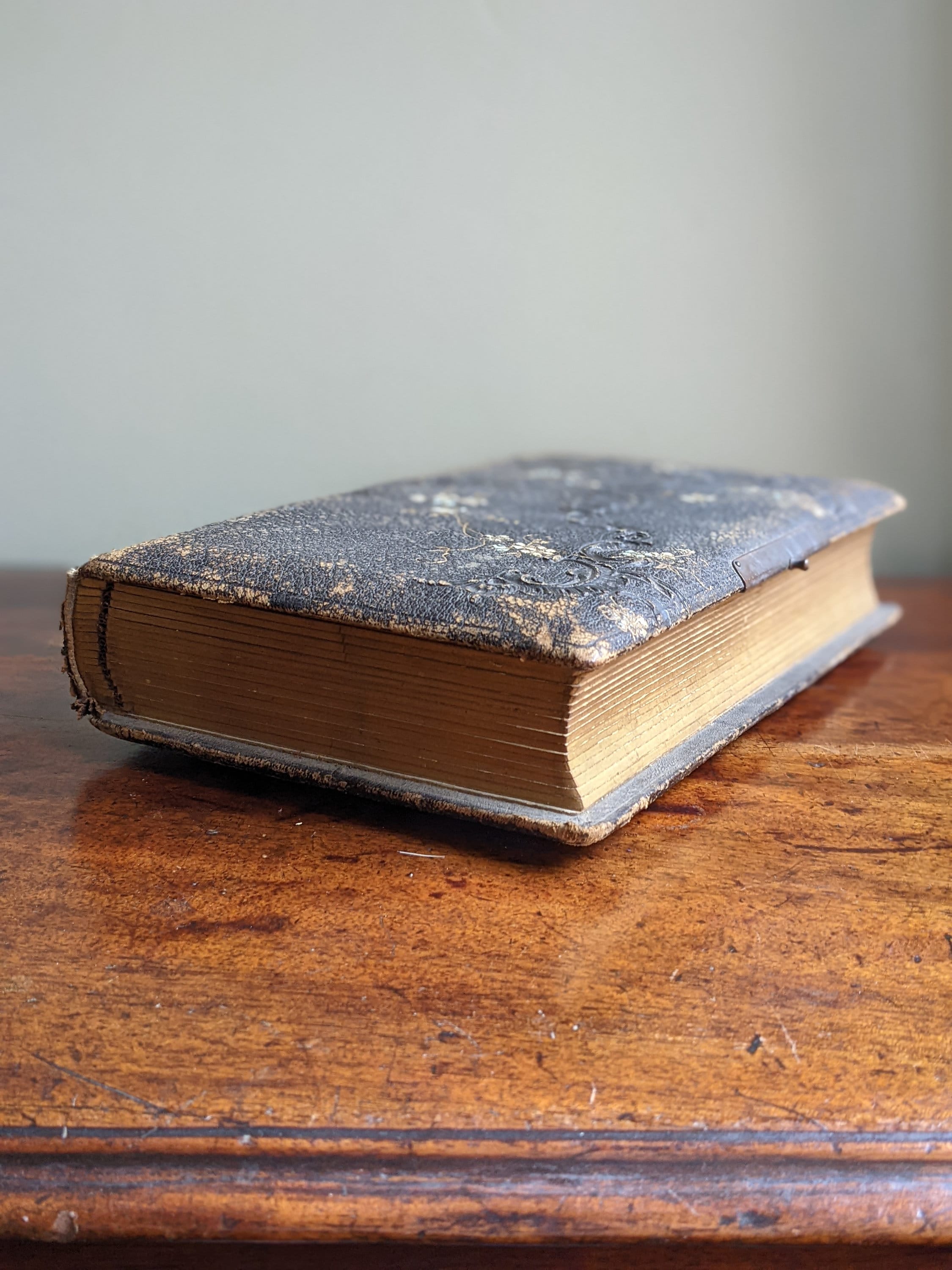The image showcases a close-up color photograph of an antique book resting on a well-worn wooden coffee table. The table, characterized by its rich brown and dark brown grain patterns and a decorative edge, displays a multitude of small dents and scratches, emphasizing its age and use. 

The book itself, approximately 12 inches long and 6 inches wide, is observed at a three-quarter view with its bottom edge facing the viewer. The cover, originally black, is significantly worn and cracked, exhibiting white splotches and brown spots indicative of shelf wear. The binding is visible and is equally worn. There's part of a metal clasp on the front cover, though the corresponding clasp on the back cover is absent. The pages, darkened to a goldish brown with age, contribute to its ancient appearance. 

Natural light enters from the right, casting soft shadows to the left side of the book. In the background, an empty, grayish-white wall with subtle shadows can be seen. The reflection of the book on the glossy surface of the coffee table adds a touch of realism to the serene indoor setting, which suggests a moment frozen in time.